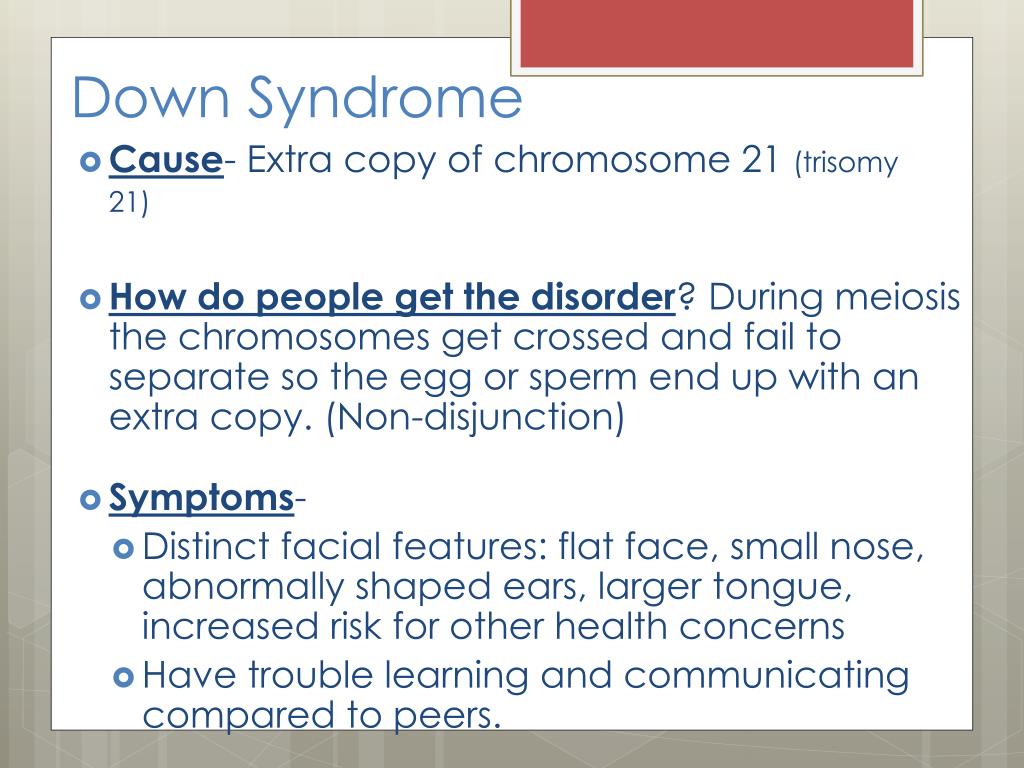A detailed and clean caption for the described image could be:

---

The top right corner of the image features a gray border. Adjacent to this border is a red circle with blue text underneath, which reads: "Trisomy 21: Down Syndrome." This section explains that an extra copy of chromosome 21 causes Down Syndrome, emphasized by the underlined text.

Below this is another circle, left unchecked, with the question: "How do people get the disorder?" Underneath, it is explained that during meiosis, chromosomes may fail to separate properly—a process called non-disjunction—resulting in an egg or sperm with an extra copy.

The image includes three bullet points outlining symptoms:
1. Distinct facial features such as a flat face, small nose, abnormally shaped ears, and a larger tongue.
2. Increased risk for other health concerns.
3. Difficulty in learning and communicating compared to peers.

The font style is mainly not bold, except for the underline, which enhances key details. The overall layout is designed to provide clear and concise information about Down Syndrome.

---